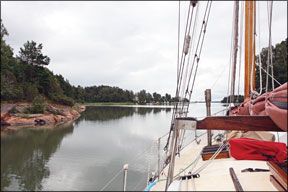This is a very small photograph taken from onboard a sailboat. The image captures a scenic view dominated by a muddy, dark-green river that stretches to a horizon almost blending with a cloudy, sunless sky. To the left, the riverbank features reddish-colored soil and is densely populated with lush, green trees whose reflections can be seen in the water, adding to the vivid greenery. The rocky shore contrasts sharply with the verdant foliage. The boat itself has distinct features, including a teak-colored deck, a prominent brown mast with elaborate rigging, and a silver railing at the front. While no sails are raised, there's a visible mauve-colored sail and a red fabric piece atop the boat's right side. The well-described mast and wood accents contribute to the detailed and authentic feel of a sailor's environment.